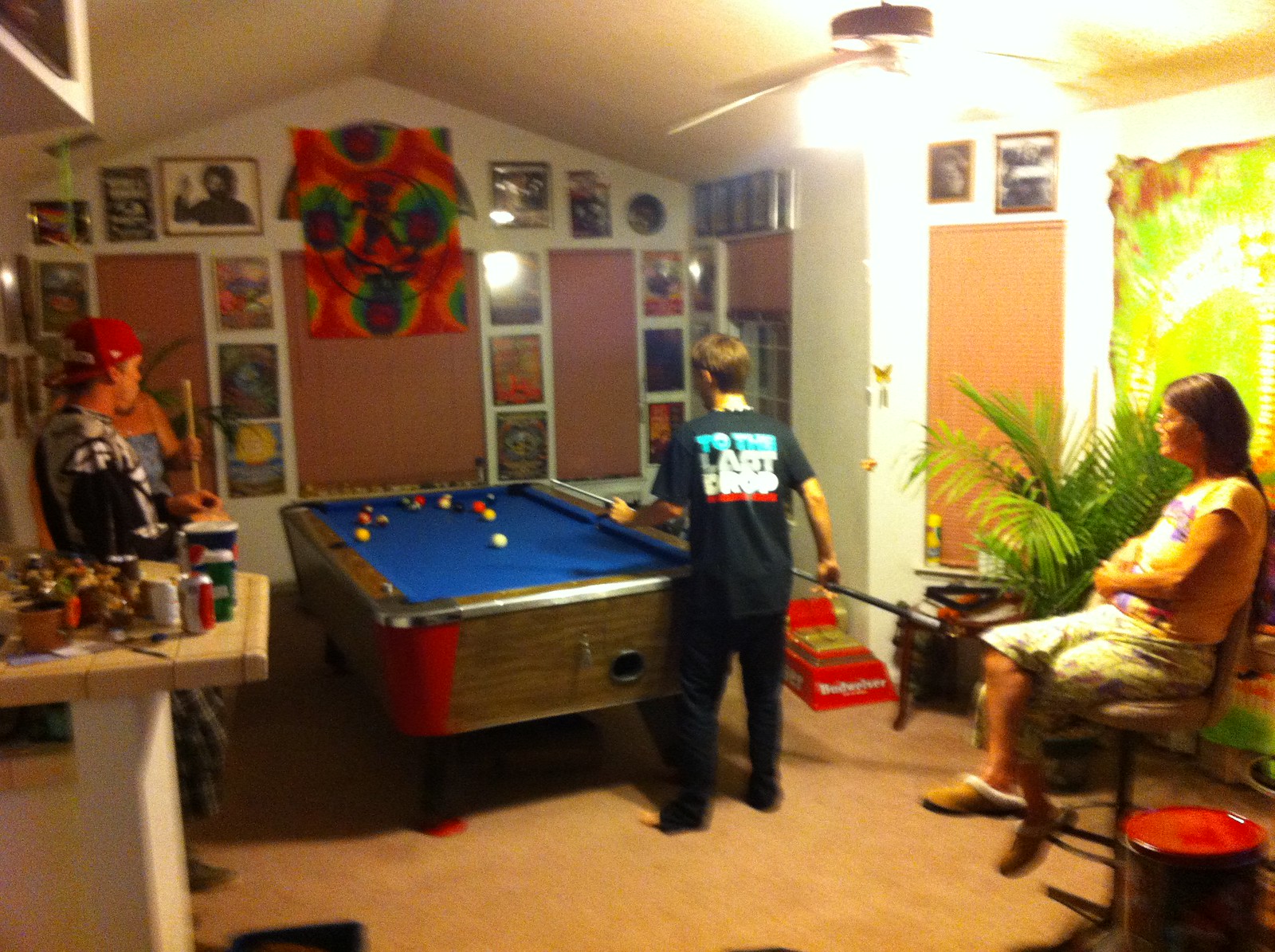The image captures a lively game room situated within a home, featuring a prominently placed pool table with blue felt and red corners. In the center of the room, three young men in their late teens or early twenties are engaged in a game of pool, with one of them aiming his shot. The young man at the table wears a black shirt that reads "to the last droid." Surrounding them are various memorabilia-decorated walls, including tie-dye tapestries and possibly Grateful Dead-related items. Framed portraits and other posters add to the room’s eclectic decor, while drapes cover the windows. 

A countertop cluttered with soda cans, bottles of beer, and assorted knickknacks is visible, reinforcing the laid-back, hangout atmosphere of the space. An older woman, dressed in slippers and glasses, sits on a high-back stool towards the right of the pool table, slightly blurred in the image, seemingly out of place among the youthful activity, like a mother supervising or joining in on the fun. There is also a plant positioned near her, adding a touch of greenery to the vibrant room. Altogether, the scene exudes a casual, familial vibe as the group enjoys an evening of pool in their game-centric living space.